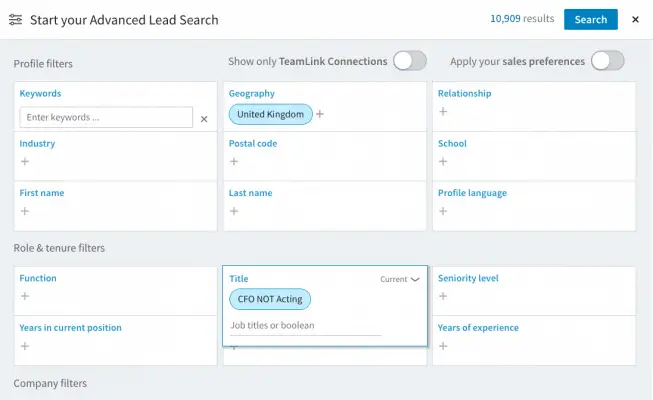The image is a horizontally-oriented rectangle featuring a structured layout designed for an advanced lead search interface. The background is pale gray, containing an organized array of individual white boxes, each holding various types of information. Above the pale gray section, set against a white background, the top-left corner displays the text "Start your advanced lead search" in black. To the right, bold bright blue text reads "10,909," followed by the word "results" in light gray. Adjacent to this, a bright blue button contains the word "Search" in white text, and a black 'X' icon is positioned to close the page.

In the upper-left quadrant of the pale gray section, the text "Profile Filters" is prominent, with an input box below it allowing filters by "Keywords," "Industry," and "First Name," all highlighted in bright blue. To the right of this, the box is labeled "Show only Team Link connections," accompanied by a toggle switch that is currently set to the 'off' position.

Beneath these sections is another white box for searching by "Geography," "Postal Code," and "Last Name." To the right, another area provides fields for "Relationship," "School," "Profile," and "Language." The interface is designed to be user-friendly, with multiple filters and search parameters, extending further down the page with additional organized information boxes.